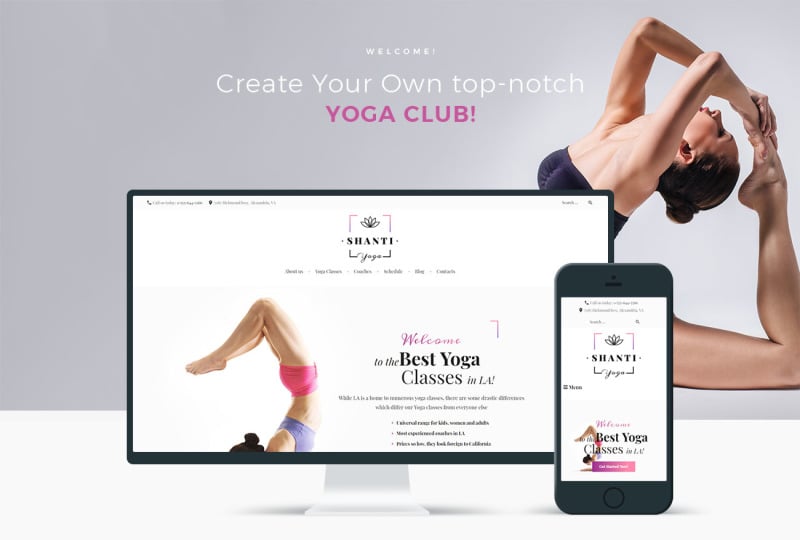This image is a detailed screenshot from a yoga website. The upper background predominantly features a shade of gray, transitioning to white towards the bottom. Prominently displayed in white text at the top is the welcoming message: "Welcome, create your own top-notch yoga club," with "Yoga Club" highlighted in pink.

On the right side of the image, a woman is captured mid-yoga pose, executing a challenging move where she bends her back and arms to reach her toe, which is raised towards her head. She is dressed in a strapless top. However, much of her body is obscured by an overlaid image of a computer screen displaying the same website.

The computer screen showcases the website titled "Shanti" with visible menu options. A depiction of a person performing a scorpion pose is also visible, accompanied by the text, "Welcome to the best yoga classes in LA," followed by additional, smaller text that is illegible. 

Adjacent to the computer, a smartphone screen mirrors the same website display, showing the "Shanti" title and "best yoga classes in LA" message. The phone appears disproportionately larger compared to the computer in this composition. The base of the computer screen is white, blending with the lower white section of the background.